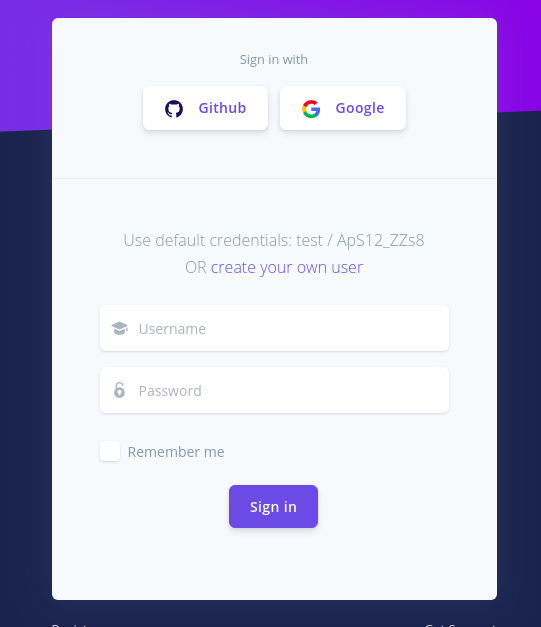A detailed screenshot of a website or app login pop-up is displayed. It is cropped to partially reveal a gradient background, transitioning from a light purple at the top to a darker purple beyond the center to the bottom. The prominent pop-up is white and centrally positioned. At the very top, the text "Sign In" is centered, followed by two horizontally aligned login options beneath it. The left box displays the 'GitHub' authentication option, while the right box offers 'Google' authentication. Both buttons feature white backgrounds with their respective logos on the left side and their names in purple text to the right.

Below these options, centered text reads, "Use default credentials: test and then a code, or create your own user," where the phrase "create your own user" is highlighted in dark purple. Following this instruction are fields for entering a username and password, accompanied by a "Remember Me" checkbox on the bottom left.

Finally, a prominent purple "Sign In" button is centered at the bottom of the pop-up. The overall layout is clean and functional, emphasizing the various sign-in options and user instructions clearly.